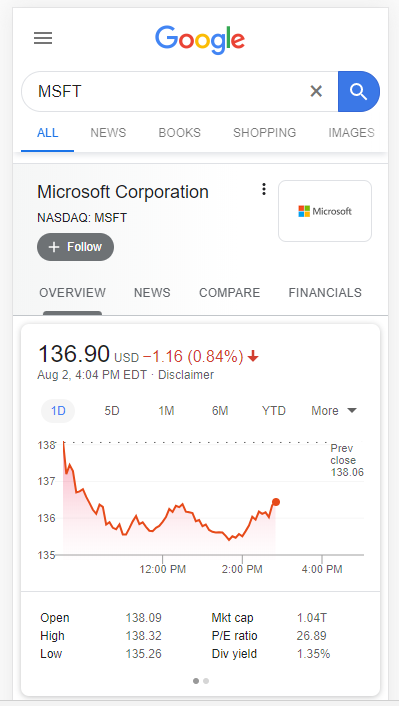The image displays a screenshot from a mobile phone, specifically showing the Google search results page for "MSFT," which is the stock ticker symbol for Microsoft Corporation on the NASDAQ stock exchange. The search results are under the "All" tab, with other tabs such as News, Books, Shopping, and Images visible but not selected. Below the search bar, there's a section dedicated to Microsoft Corporation, with its NASDAQ symbol (MSFT) prominently displayed. The section includes the Microsoft logo on the right side.

Further down, the screen shows several sub-tabs including Overview, News, Compare, and Financials, with the Overview tab currently selected. The Overview tab provides detailed financial information, including the stock price listed in US Dollars at $136.90, as of August 2nd (the year is unspecified). The data appears to be reflecting the one-day trading statistics, with a line graph displaying stock performance throughout the day. The graph indicates that the time is approximately just before 3 PM and that the stock price is trending upwards.